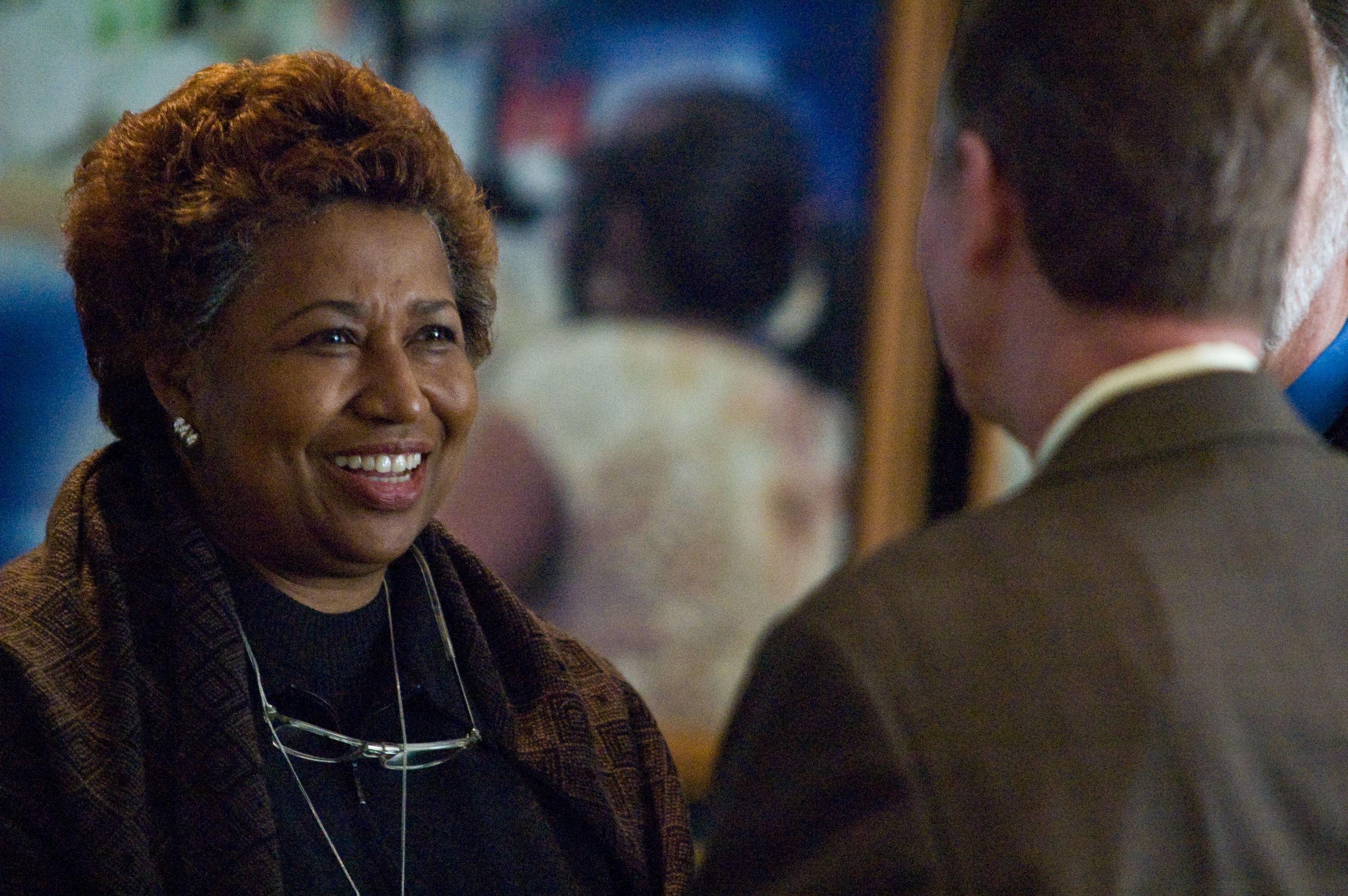The horizontal rectangular image captures an engaging scene between two people. On the left is an African-American woman with reddish-brown hair, including black roots. She has a radiant smile showcasing her top front teeth and wears triple pearl earrings. Her glasses, which have gray front frames, dangle around her neck on top of a black shirt with a zipper just beneath them. She’s wrapped in a bronze-colored shawl with a maroon and brown pattern. The man on the right, whose face isn’t visible, is a white male with short brunette hair. He is dressed in a brown business jacket over a light-colored shirt with a visible collar. Behind them, a mirror reflects another individual with dark hair and a light-colored sleeveless blouse. Additionally, another reflection, possibly of a person with silver hair in blue attire, can be spotted in the upper right corner, adding layers to this vivid and detailed portrayal.